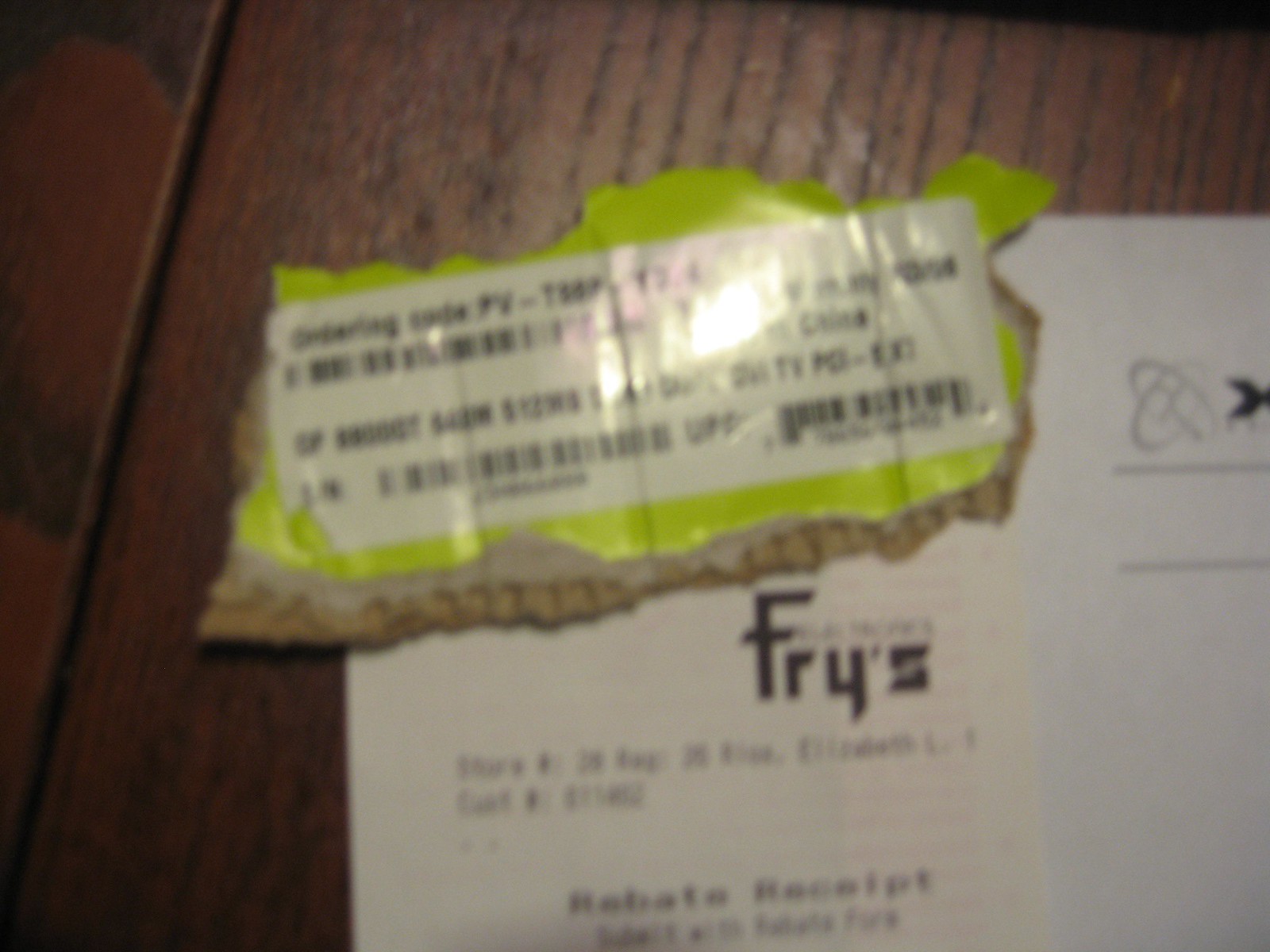A detailed image of a piece of paper on a wooden table. The paper prominently displays the word "Fry's" in large, bold, black letters, with the spelling "F-R-Y-apostrophe-S". Below this heading, in much smaller and hard-to-read print, the words "rebate receipt" are visible, indicating that this document is a receipt for a rebate. The paper also includes a return address, however, this section appears partially torn. The document is affixed to a piece of cardboard, which seems to have been ripped from a larger box, visible in the upper left corner. The wooden table beneath features clearly defined and visibly separated planks, with the wood grain and lines accentuating the rustic texture of the surface.